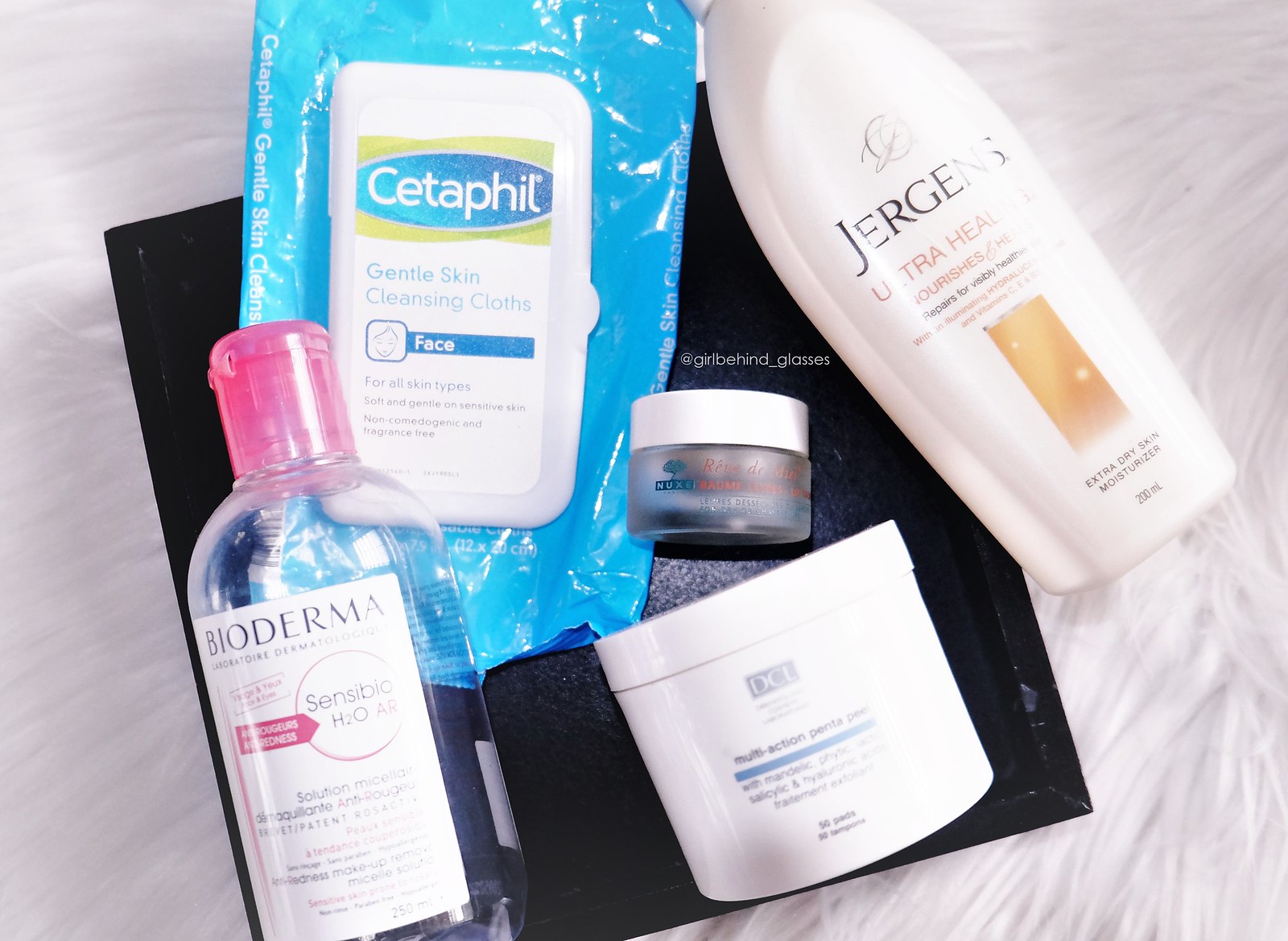This photograph showcases an arrangement of health and beauty products set against a clean, white background. The backdrop features a textured white cloth, providing a soft and elegant base for the display. At the center, a black square tray sits atop the cloth, serving as a tidy organizer for the items.

On the tray, there is a bottle of Juergens Ultra Healing Lotion prominently placed. Beside it, a small jar containing a dark cream can be seen, revealing its contents through the clear glass. Below this jar is another container, a white bottle with partially visible branding that reads "DCI," suggesting it is a type of face or body cream.

To the left of the tray is a clear bottle labeled Bioderma, indicating that it is a facial cleansing solution, presumably for sensitive skin, as suggested by the partial reading of "Sensible H20."

Above these products lies a pack of Cetaphil Gentle Skin Cleansing Cloths, completing the array of skincare essentials. The overall composition is thoughtfully arranged, highlighting each product distinctly while maintaining an organized and aesthetically pleasing presentation.